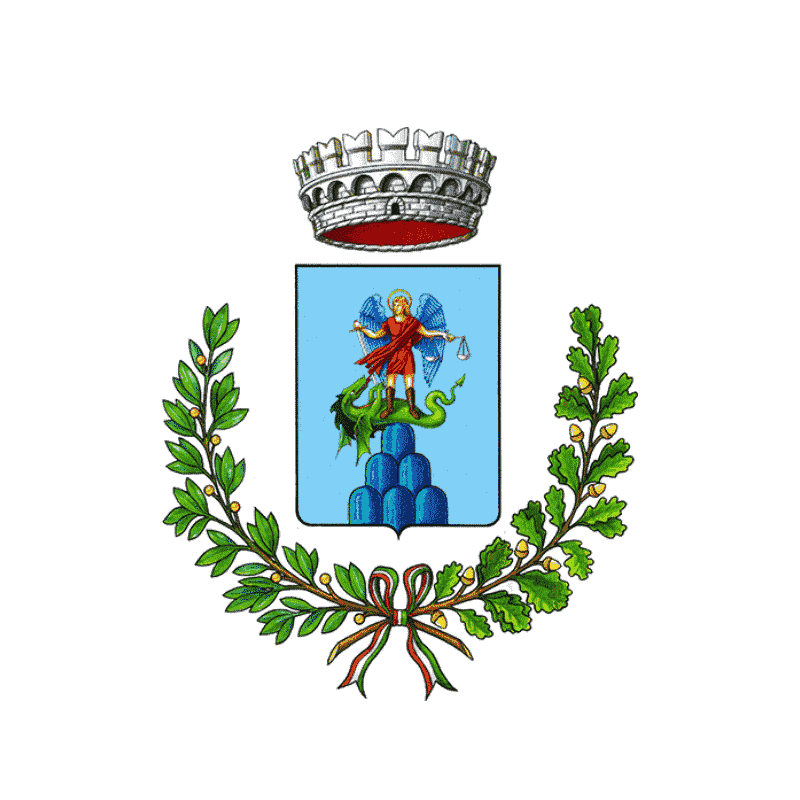This intricate illustration appears on a white background and resembles a well-designed coat of arms, possibly also imagined as a logo or a shield. Centered in the image is a blue rectangular section portraying a woman depicted as an angel with blue wings and a red dress, holding a sword and a set of scales. She stands triumphantly over a green dragon situated on a blue mountain. Floating above this scene is a silver crown with castle-like features and a red border. Surrounding the lower half of the rectangle is a wreath composed of green leaves, berries, and acorns, all tied together with a red, white, and green ribbon.